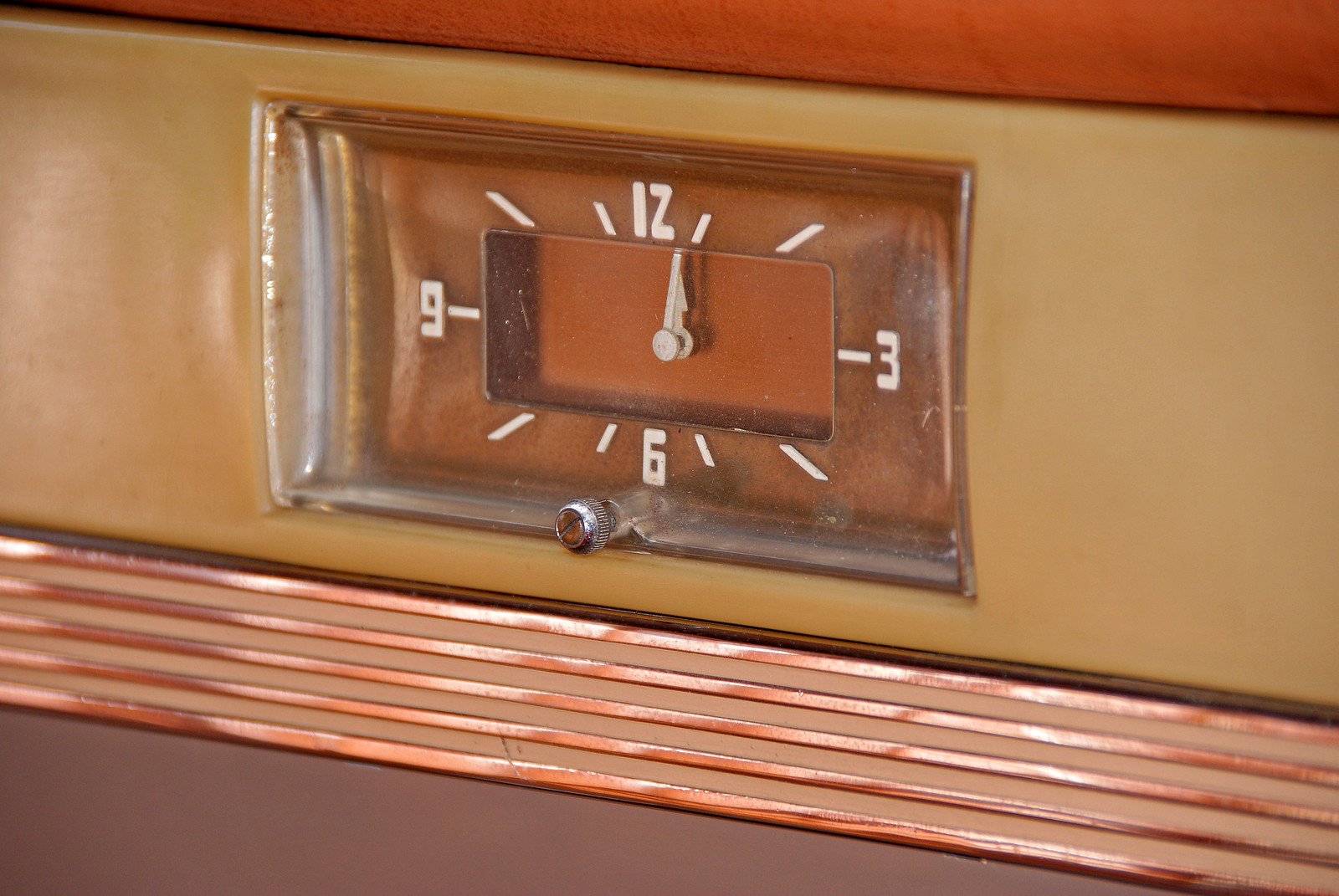The photograph captures a close-up view of a vintage analog clock embedded in the dashboard of an older vehicle, possibly a 1950s Cadillac. The clock is small and rectangular with a protective glass cover, secured by a visible screw at the lower edge. The face of the clock, set to 12 o'clock, displays only the numbers 12, 3, 6, and 9 in white, with the hands nearly identical in size. The clock is nestled in a tan-colored leather section of the dashboard, flanked by wood grain strips above and below it. These wood strips are interspersed with gold accents, adding to the retro aesthetic. The dashboard itself appears to be made of vinyl, with varying textures and colors visible, including green, red, and tan elements.